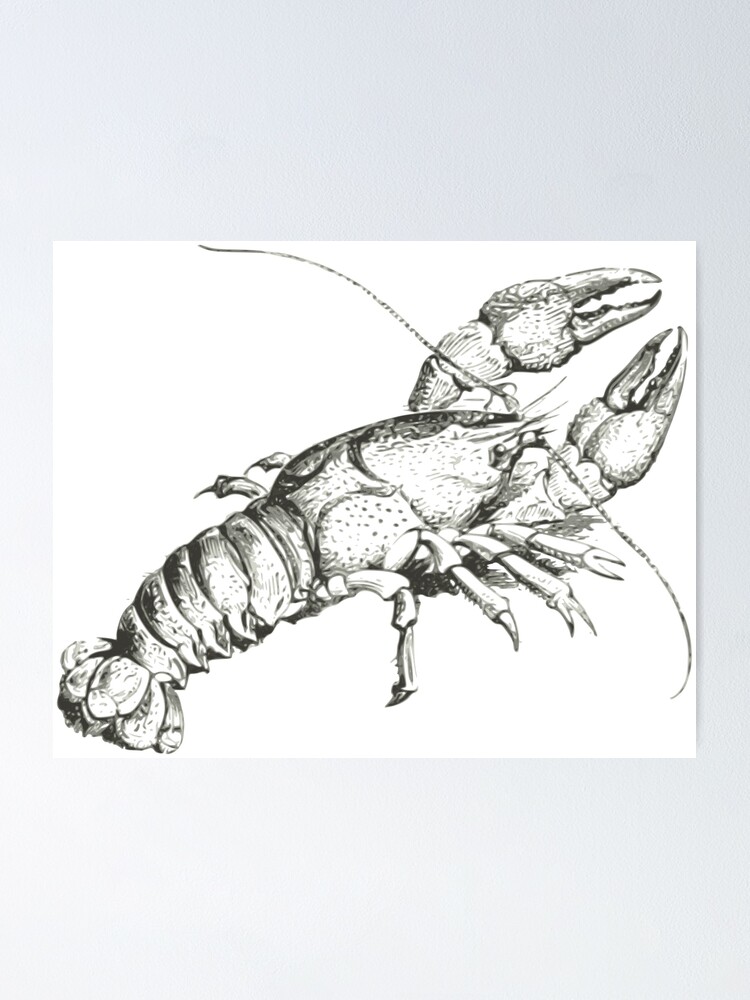The image depicts a detailed, black and white illustration of a lobster. The lobster is positioned from left to right, with its tail situated in the bottom left corner and its large, slightly open claws occupying the top right. The claws are prominent and suggestive of considerable power, with strong arms connecting them to the body. The lobster's body, which has an almond-like shape, is adorned with black spots and features a hard, crusty shell. Its long antennas stretch nearly the length of its body on both sides. The legs are visible, with six clearly seen—four on the right side and at least two on the left. The tail, approximately half the length of the body and ribbed with petal-like segments at the end, accentuates the crustacean's distinctive form. The illustration is set against a lightly gray gradient background, darker at the top transitioning to nearly white at the bottom, and is presented as a straightforward, uncolored sketch, rendered in either pencil or pen.